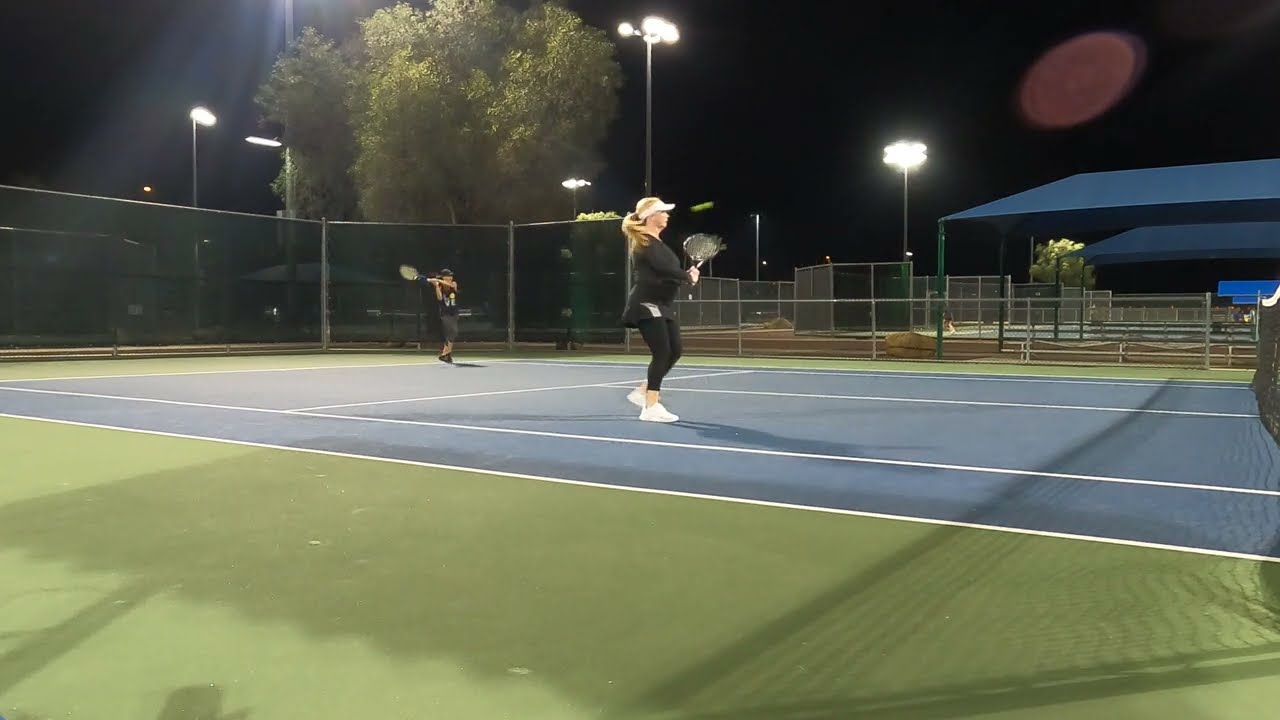This is a detailed nighttime photograph of an outdoor tennis court, illuminated by tall stadium lights. The court's surface is blue, with green on the sidelines and the overhead sky shrouded in darkness. The photograph captures a woman standing prominently in the center, dressed in a black shirt, black pants, and white tennis shoes. She is mid-movement, holding a tennis racket up, her blonde hair captured in motion. She also sports a white visor. Slightly behind her to the left stands another figure, possibly male, in a black shirt and dark grey pants, also holding a racket in a position ready to strike. The court is surrounded by fencing, with visible trees and another awning area, suggesting a well-structured setup for either play or events. A portion of the white-topped tennis net is visible on the right side of the image, dividing the court. In the distant background, there appears to be a blue awning and a distinct red orb, which might be a light flash or the moon.